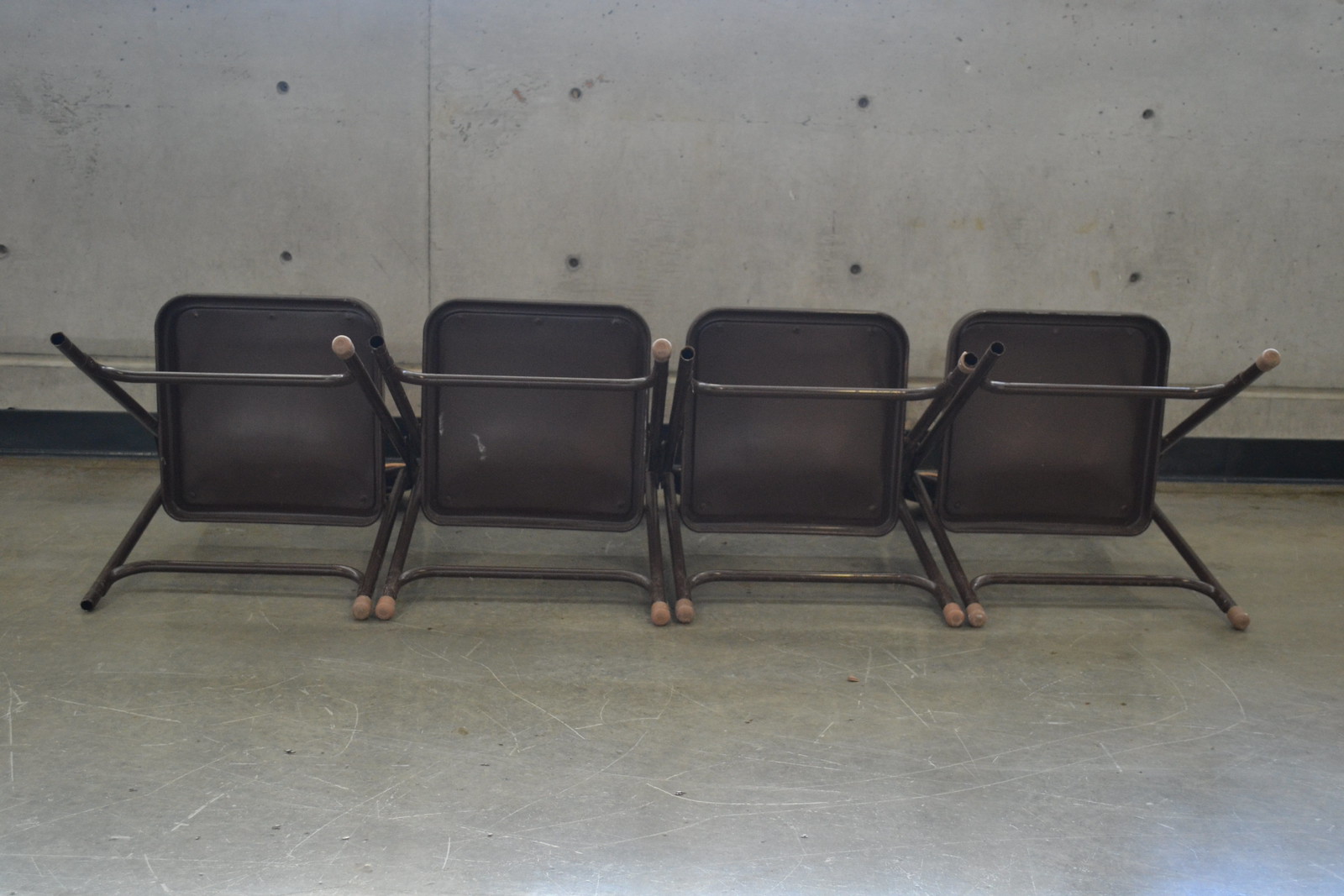This photograph, taken indoors against a plain concrete wall with visible bolt holes, shows four metal folding chairs laid on their backs in a row on a scuffed gray cement floor. Each chair, a brownish-gray or smoke-gray color, features square seats with legs formed by V-like structures connected by a supporting bar. Notably, all chairs have varying degrees of missing rubber or tan caps on their legs. You can see into the hollow legs where these caps are absent. One chair has a distinct white streak on the bottom of its seat, and there are visible rough spots on the connecting bars of some chairs. The scene highlights the uniformity and wear of these metal chairs in a stark, utilitarian setting.